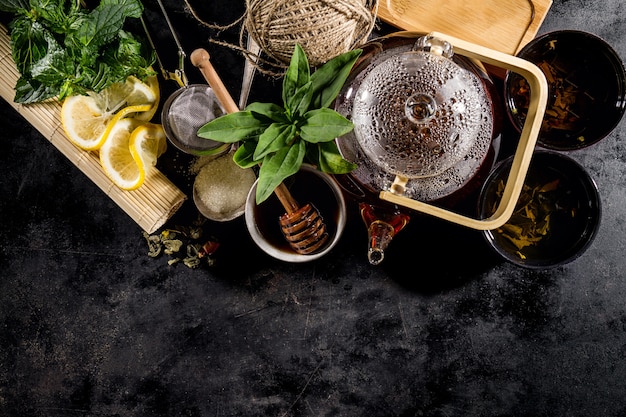This is an overhead shot featuring a meticulously arranged tea-making station set against a black marble or stone surface. In the top two-thirds of the image, laid out from left to right, there's a sushi-rolling mat, fresh mint leaves, and lemon slices, some of which are in a yellow cup and others are folded in half. Adjacent to these, a mesh strainer for tea is present. Moving right, there is a clear glass teapot filled with amber liquid, showing condensation on the inside. Above the teapot, a ball of twine is placed, and below it, a honey dipper. Slightly down and to the right, a silver pail contains a long honey stick, and next to it is a silver pot of water. Further to the right, two small black bowls are filled with tea leaves or herbs, categorized into orange and yellow varieties. Completing the setup, additional green plants and leaves are scattered around, contributing to the rustic, natural aesthetic of the tea-making station.